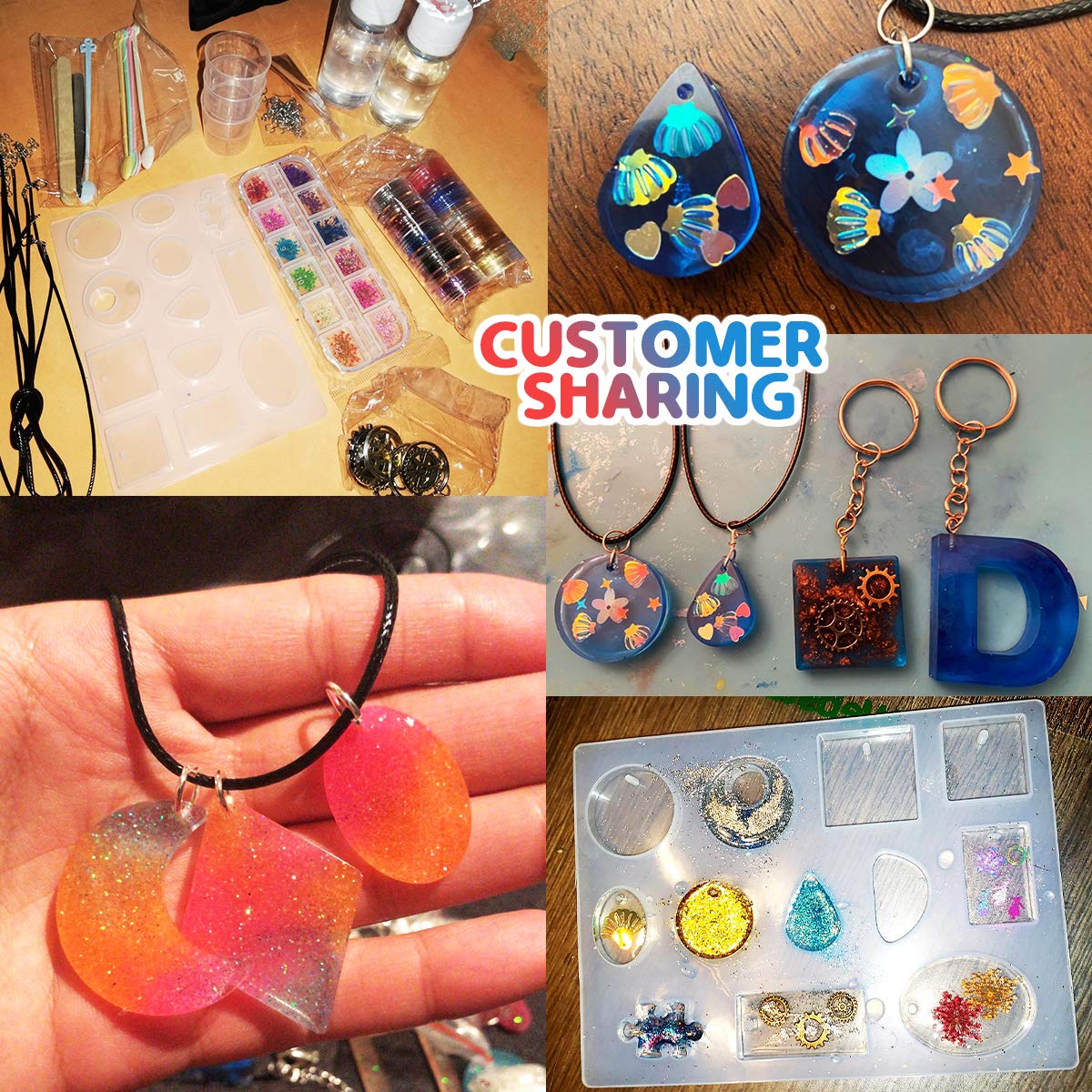The image is a rectangular collage composed of five different photographs that showcase various components and tools for acrylic jewelry making. The collage is equally divided on all four sides, with the photographs differing in size. 

In the top left photograph, a white tray filled with various shapes such as ovals and squares is placed on a flat yellow surface. Accompanying the tray, there are additional supplies including a bag of glitter and beads, rolls of fabric, spools of rope likely intended for necklaces, Q-tips, plastic cups, and two clear plastic bottles.

The bottom left photograph displays stones in shades of pink and orange, intricately attached to wires, presumably for decorative purposes or keychain making. 

On the right side of the collage, the three photographs continue to highlight the array of available materials and tools. The photographs include keychains and other decorative items, further emphasizing the versatility of the jewelry making kit.

In the middle of the collage, a text reads "Customer Sharing" in vibrant red and blue colors, bringing attention to the collaborative and community aspect of the craft.

The collage collectively illustrates the ample components provided in the jewelry making kit, encouraging creativity and showcasing the potential outcomes one could achieve using the materials.